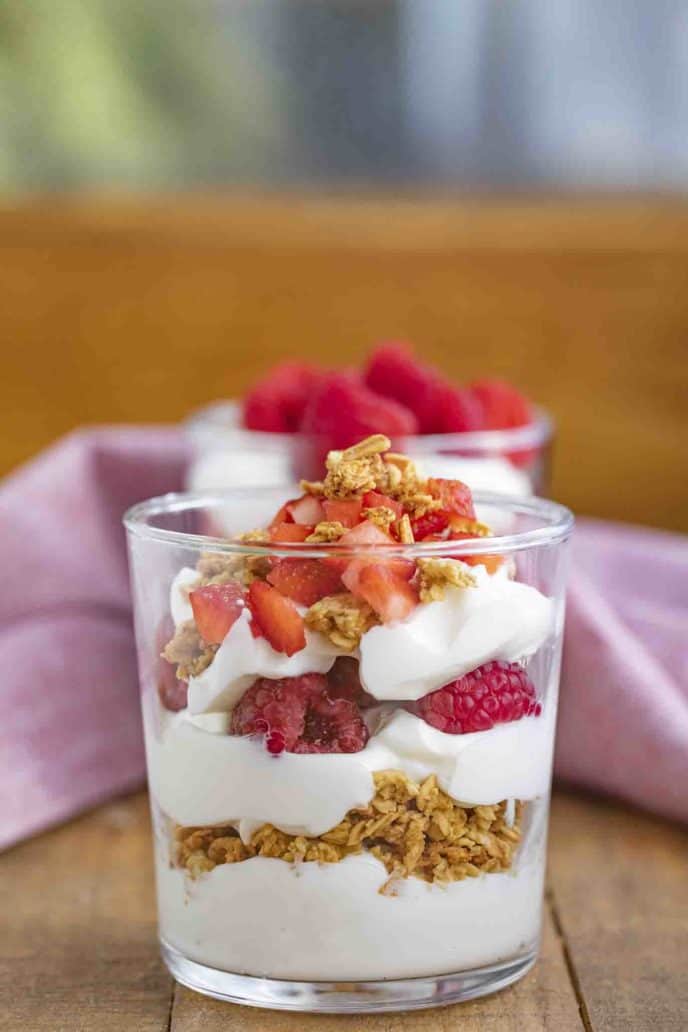This photograph captures a close-up view of two glass cups filled with a beautifully layered dessert, potentially a fruit parfait. The cups are placed on a light brown, rustic wooden table. The focal point is the first cup, which is prominently detailed, displaying distinct layers of whipped cream or yogurt, brown granola, vibrant red raspberries, and thinly sliced strawberries topped with nuts. The second cup, positioned slightly behind the first, appears to contain similar contents but is more blurred due to the shallow depth of field.

Behind the second cup, a pink napkin or paper towel stands out, adding a splash of color to the composition. The tightly framed photograph makes the background indistinct, but hints of a light brown or green object are visible in the top left corner, alongside a faintly visible white wall on the right. The subtle details of the background, including possibly another window or wall, remain beautifully blurred, keeping the focus on the intricate layers of the parfait in the foreground.

This image artfully captures the textures and colors of the dessert, making it not only visually appealing but also indicative of a delicious snack or breakfast option, meticulously crafted and presented.